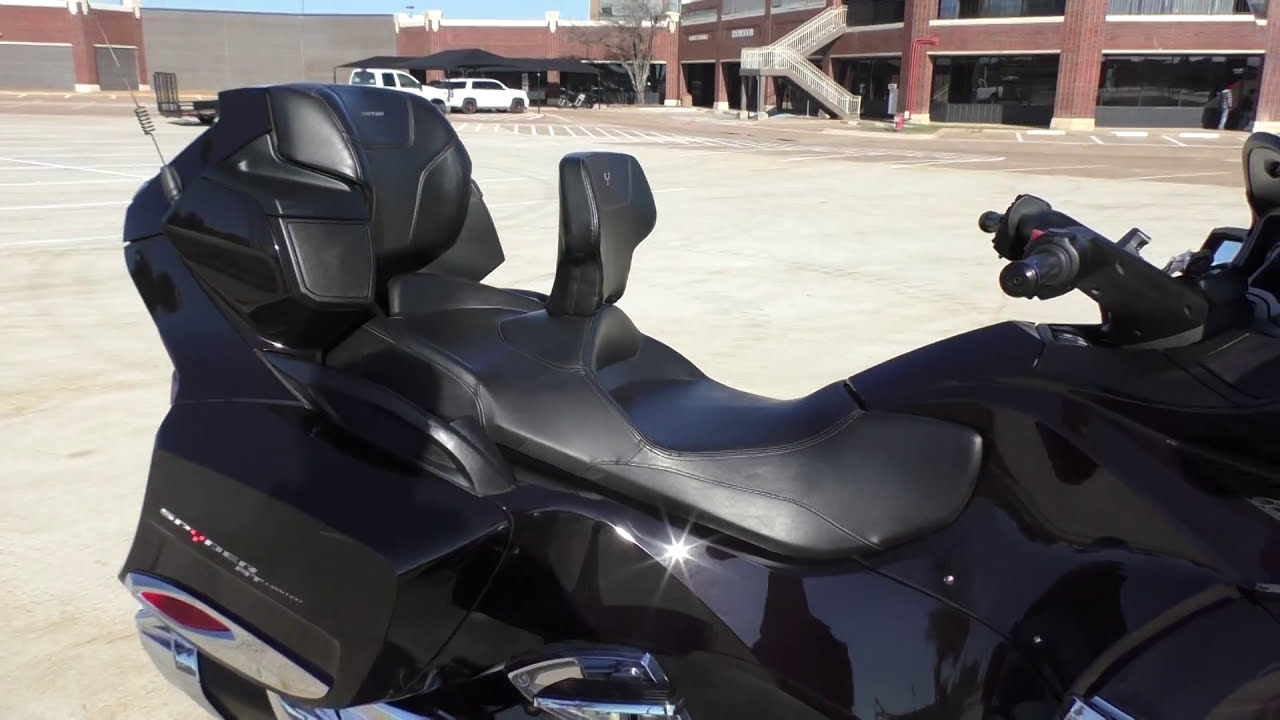In this image, a sleek black motorcycle with chrome detailing is prominently displayed in the foreground, its glossy surface catching the light. The motorcycle appears to have dual seats and prominent handlebars, though the front wheel is out of the frame. It is parked in a spacious concrete or dirt lot. Surrounding the lot, there are several buildings, primarily made of red brick. One of these buildings has white railings leading up to a second floor, which suggests it could be part of a strip mall or a factory complex. The area includes a couple of white vehicles—a SUV and a truck. To the left, there are large metal garage doors, and in the background, the windows of the brick buildings are dark, contributing to an unfinished or industrial aesthetic. The sky is a light blue, visible above the buildings.